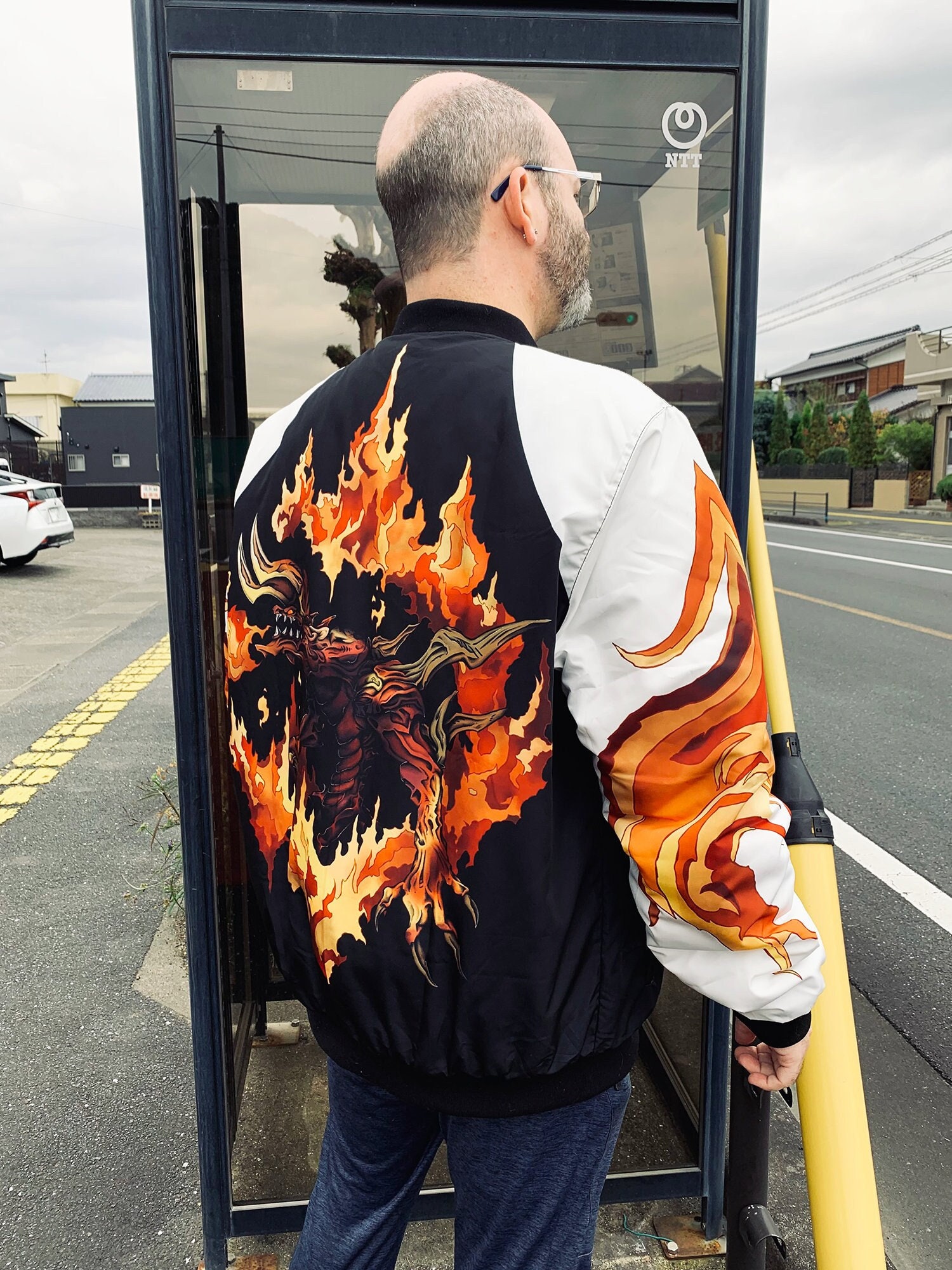The image captures the back of a Caucasian man with thinning black hair and a thin black beard with a gray chin. He is standing at a bus stop, indicated by the glass booth in front of him. The man is wearing a distinctive jacket with a black body and white sleeves. On the back of the jacket is an elaborate design featuring a dark red demonic dragon with twisted brown horns and long, sharp brown claws. This dragon is encircled by vibrant flames in shades of red, orange, and yellow. The sleeves of the jacket are adorned with similar flame patterns, creating the impression of a dragon's tail wrapping around them. The man is also seen wearing blue jeans or sweatpants. The surroundings seem to include some houses, adding context to where this scene is taking place.